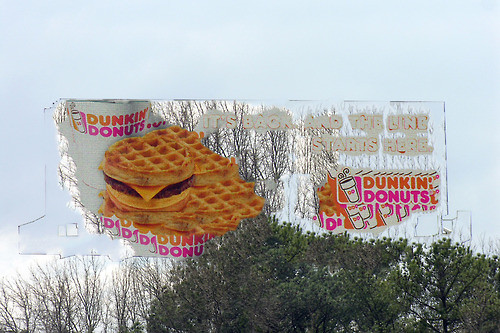The image showcases a vibrant Dunkin' Donuts sign prominently displayed above a cluster of trees. At the bottom right of the image, dark green leafy trees are visible, while the left side features barren trees with vertical branches devoid of leaves. The sign itself highlights a promotional message with white text stating "It's Back! The Line Starts Here," accented with a touch of orange. On the bottom right of the sign, the word "Dunkin'" appears in bright orange, followed by "Donuts" in bold pink, accompanied by a coffee cup logo split into orange and pink hues with a white cup outline. To the left of the text, an enticing image of sandwiches, featuring sausage and cheese between waffle buns, is displayed alongside a white Dunkin' Donuts cup. Above the sign, the serene sky stretches out in a light blue expanse.